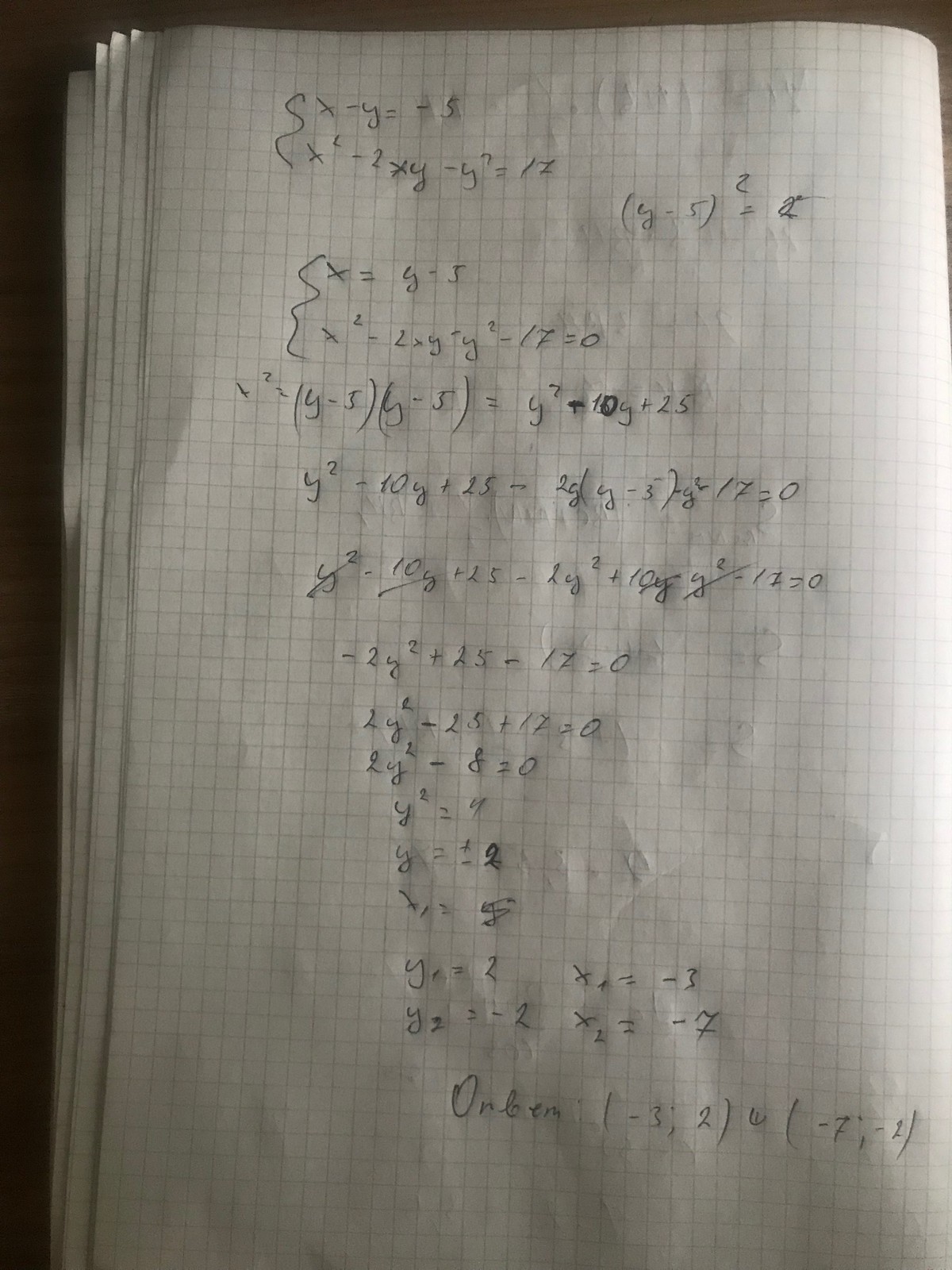The image showcases a math equation written on graph paper, which resides in a graph paper notebook with the edges of the notebook visible on the left-hand side. The background beyond the paper is black, providing a stark contrast to the writing. The equation itself appears to be written either with a mechanical pencil or a fine black pen, indicated by the consistent and dark lines. At the very top of the page, there is a squiggle resembling a parenthesis, followed by the equation "X - Y = -5."

The handwriting is somewhat difficult to read due to its messy and hurried nature, with irregularities and extra turns that suggest it was written quickly. The writing occupies most of the page, extending almost to the bottom and is roughly centered rather than aligned to the left. Notably, about a third of the way down the page, there is a visible correction where the writer traced over the letters multiple times to fix a mistake. Overall, the script lacks uniformity and neatness, contributing to its challenging legibility.